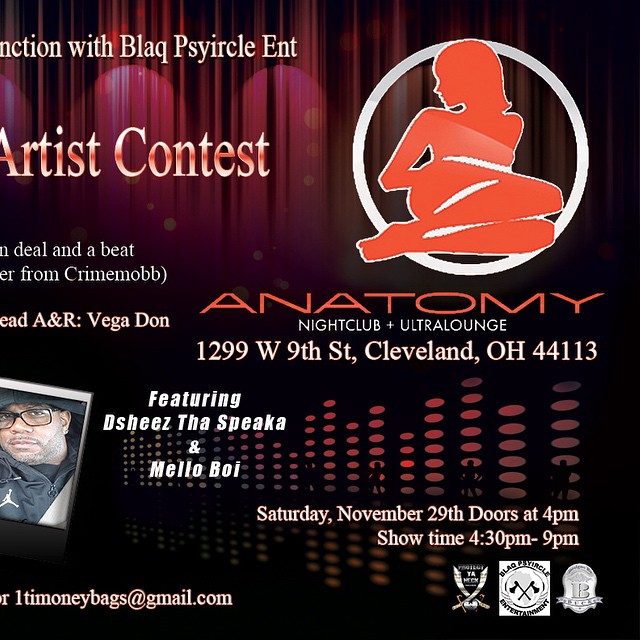The image depicts a promotional poster for an event titled "Artist Contest" at Anatomy Nightclub and Ultra Lounge, located at 1299 West 9th Street, Cleveland, Ohio, 44113. The background features a stage-like setting with dark red and black curtains. There is text at the very top with partially visible letters "N-C-T-I-O-N," and more illegible text, followed by "B-L-A-Q" and "P-S-Y-I-R-C-L-E" in black. Prominently showcased are large white letters with red accents reading "Artist Contest," and an orange silhouette of a reclining woman with a white circular border positioned in the upper right corner.

Below, in bold red letters, the word "Anatomy" is displayed along with the venue details: "Nightclub plus Ultra Lounge." Further down, the event details include the performers' names: Desheez, Tha Spica, and Mellow Boy, with the address "1299 West 9th Street, Cleveland, Ohio, 44113." The event date is presented in the lower right-hand corner as "Saturday, November 29th," with doors opening at 4 p.m. and the show running from 4:30 to 9 p.m. Additionally, there is an image of an African American man, Desheez, looking directly at the camera, located in the bottom left corner of the poster. The overall color scheme includes shades of red, purple, black, white, grey, and orange, giving the poster a vivid and dynamic appearance.